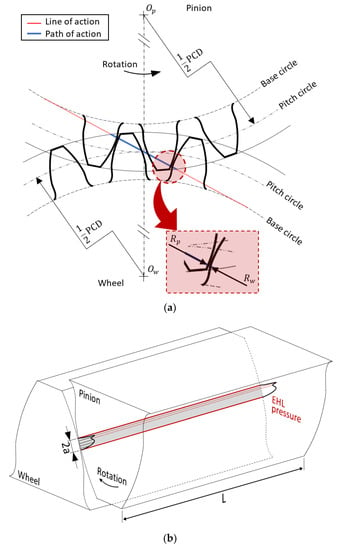The image is a detailed scientific schematic depicting the dynamics of a mechanical process involving pinion and wheel rotation. In the top left, a red line marked "line of action" and a blue line labeled "path of action" indicate key movement trajectories. The top right section includes the term "pinion" and a dashed horizontal line with an accompanying rotation arrow. Several delineations for "base circle" and "pitch circle" intersect in a complex pattern, illustrating the relationship between different mechanical components. Below, two distinct figures showcase the rotational mechanics in both 2D and 3D perspectives; these figures are separated by a central bar and composed of transparent blocks labeled "pinion," "wheel," "rotation," and "EHL pressure." The inclusion of mathematical notations, such as "one half PCD," suggests an intricate analysis of the mechanism's function.